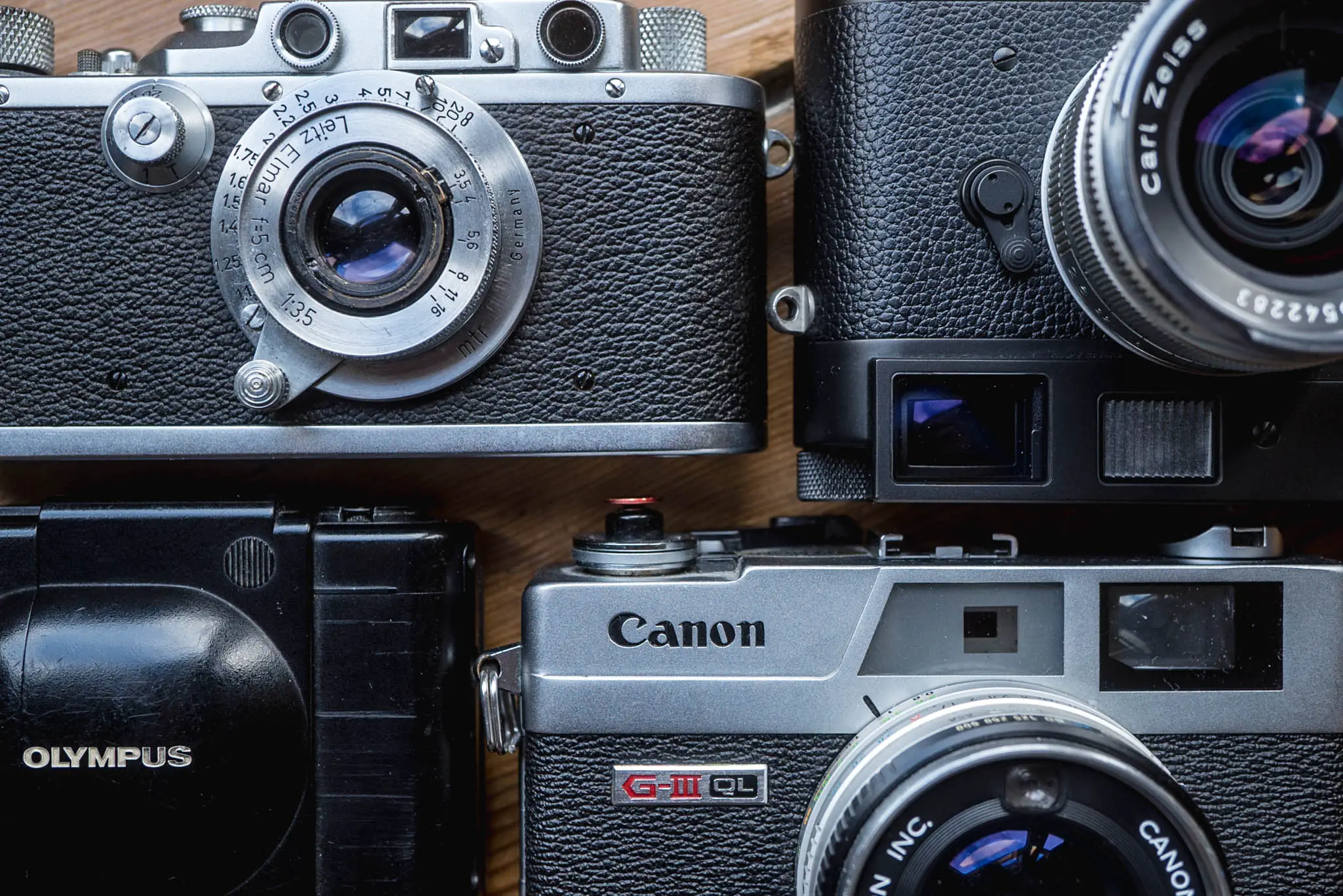The photograph captures a detailed close-up of four vintage cameras, artfully arranged on a brown wooden table. Each camera exudes a nostalgic charm, adorned with a mix of classic black and silver hues, devoid of any vibrant colors. The iconic brands Canon, Olympus, and Carl Zeiss mark the lenses, with one camera displaying text that suggests it might be German. Three of the cameras showcase the traditional single-lens reflex (SLR) design, boasting a textured grip that hints at their rugged use. In contrast, the fourth camera, an Olympus model, stands out with its smooth, compact design and a sliding front cover. The cameras, partially cropped and fitted together like puzzle pieces, create a curious scene where these once cutting-edge devices are themselves the subject of modern photography, lying against the textured backdrop of the wooden surface.